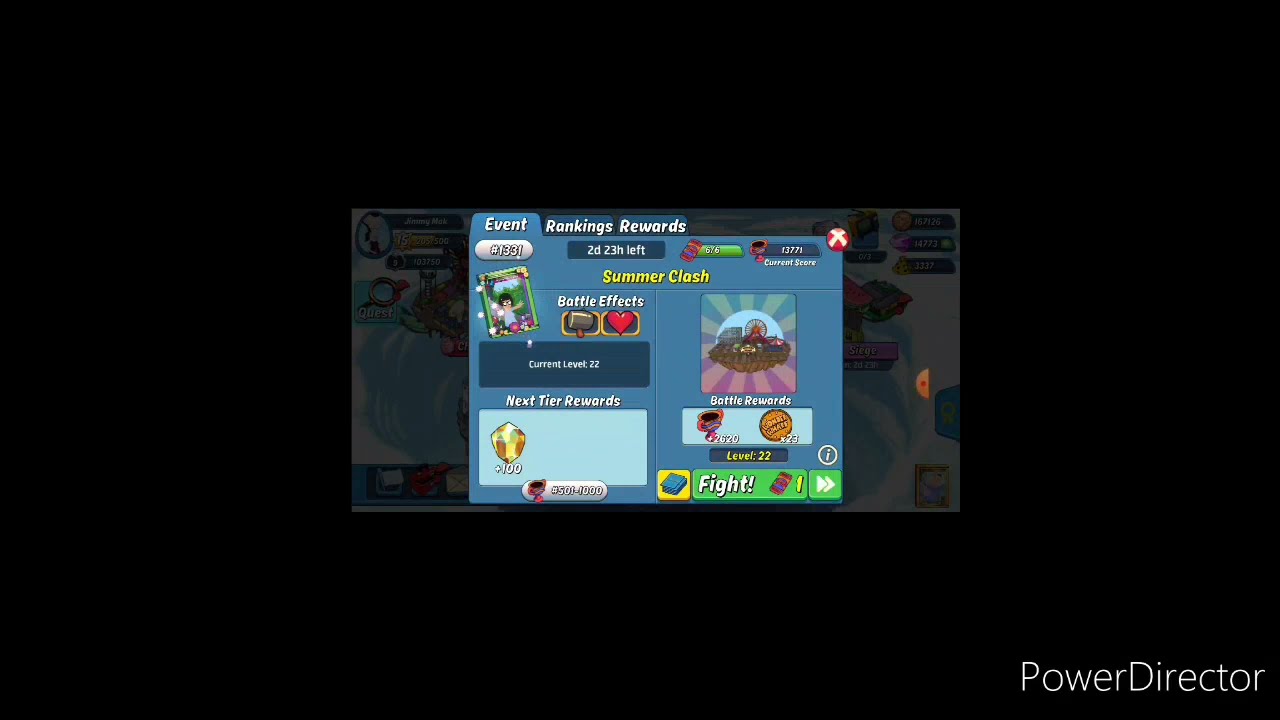This image captures a screenshot from a video game displayed on a computer monitor or laptop. The screen features a predominantly black background, with the bottom right corner marked by the text "PowerDirector." The focal point of the image is a central blue tabbed pop-up, reminiscent of a folder index, labeled with the sections "Event," "Rankings," and "Rewards." The "Event" tab is currently selected, revealing various game elements. 

At the top of the pop-up, there is a notification that reads "2 day, 23 hour left," accompanied by a green button and several icons, including a hatchet and a heart. The screen also displays a yellow banner labeled "Summer Clash," and nearby, the words "Battle Effects" can be seen. There's a character portrait on the left side, with stairs visible in the background at the top corners, indicating the gaming environment partially obscured by the pop-up. At the bottom of the event section, there's a "Fight" button, alongside various other buttons and symbols, including a UFO-like icon with rays.

Additionally, a numerical identifier "1331" is displayed on a small button, and various other icons, including diamonds and colorful shapes, are scattered across the interface. The overall appearance suggests an active game interface with multiple interactive elements and status indicators, conveying an ongoing event within the game.